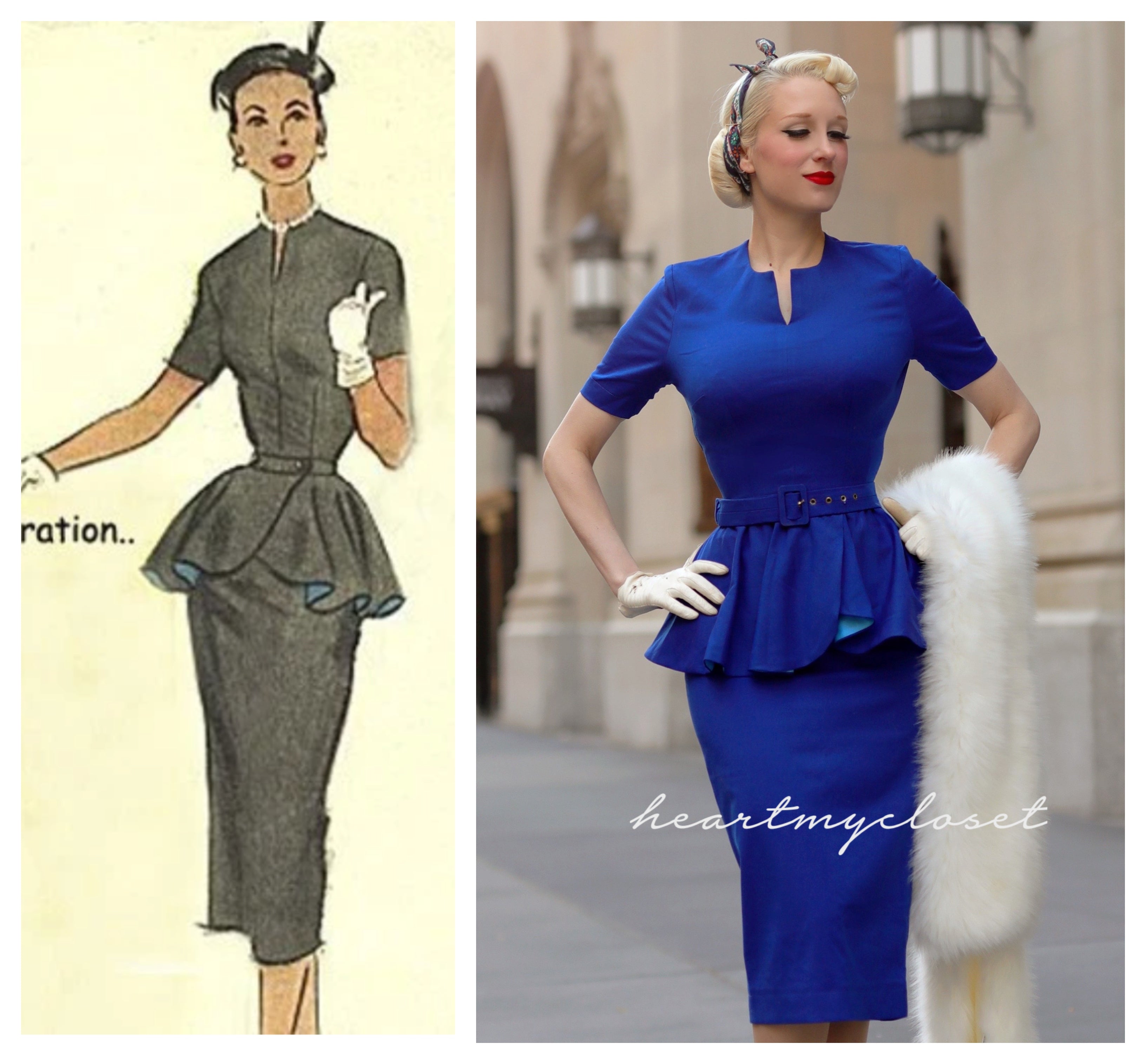The image is a dual composition, with a hand-drawn illustration on the left side and a photograph on the right. The left-hand drawing features a woman with dark, short hair, adorned in a stylish green dress paired with white gloves and a white necklace. On the right, the photograph depicts a Caucasian woman standing on a sidewalk in front of a beige or brown building. Her hair, styled impeccably and secured with a multicolored hairpin, contrasts with the drawing as she has blonde or white hair. She dons a vibrant cobalt blue dress with a blue belt accented with brass divots, along with a dark blue skirt complemented by a lighter blue underside. Matching the drawing, she wears white gloves and drapes a luxurious white mink shawl over her right arm. With her eyes closed and hands on her hips, she exudes elegance, emphasized by her red lipstick. Below the photograph, the words "Heart My Closet" are inscribed in cursive script, suggesting that the depicted attire is a real-life version of the illustrated design from the left, capturing the imaginative transition from art to reality.